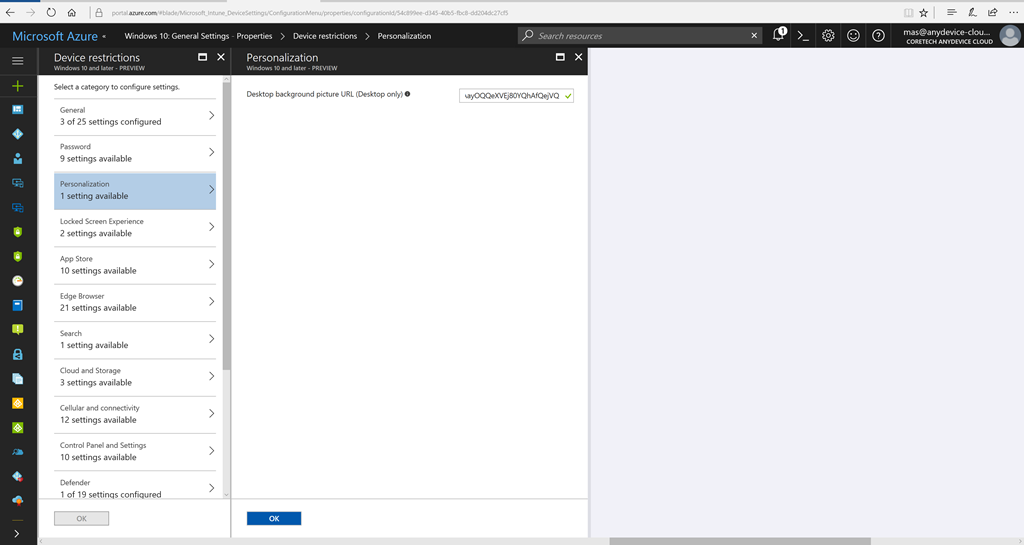This detailed caption accurately captures the content and appearance of the web page in the image:

"The image depicts a detailed view of a Microsoft Azure configuration web page, presented in a clean design dominated by white, black, and blue hues. At the top of the browser window, familiar icons such as the lock, home, refresh, and back buttons are visible, indicating the page is secure. The star icon for adding to favorites is also present. 

A prominent black banner features the 'Microsoft Azure' text in blue. Below it, various sections related to Windows 10 are displayed, including General Settings, Properties, Device Restrictions, and Personalization. 

A gray search bar lies beneath this area, flanked by notification icons, a cheerful emoji, and a profile button. To the left, a panel labeled 'Device Restrictions' provides navigation options, featuring a series of functional icons: a green plus sign, a blue square, a blue diamond, and a profile button. Other notable icons include green shields, a blue lock symbol, and a partially red cloud icon. The main content area exhibits tabs that guide users through different configurations and settings, offering a comprehensive interface for managing device and system properties."